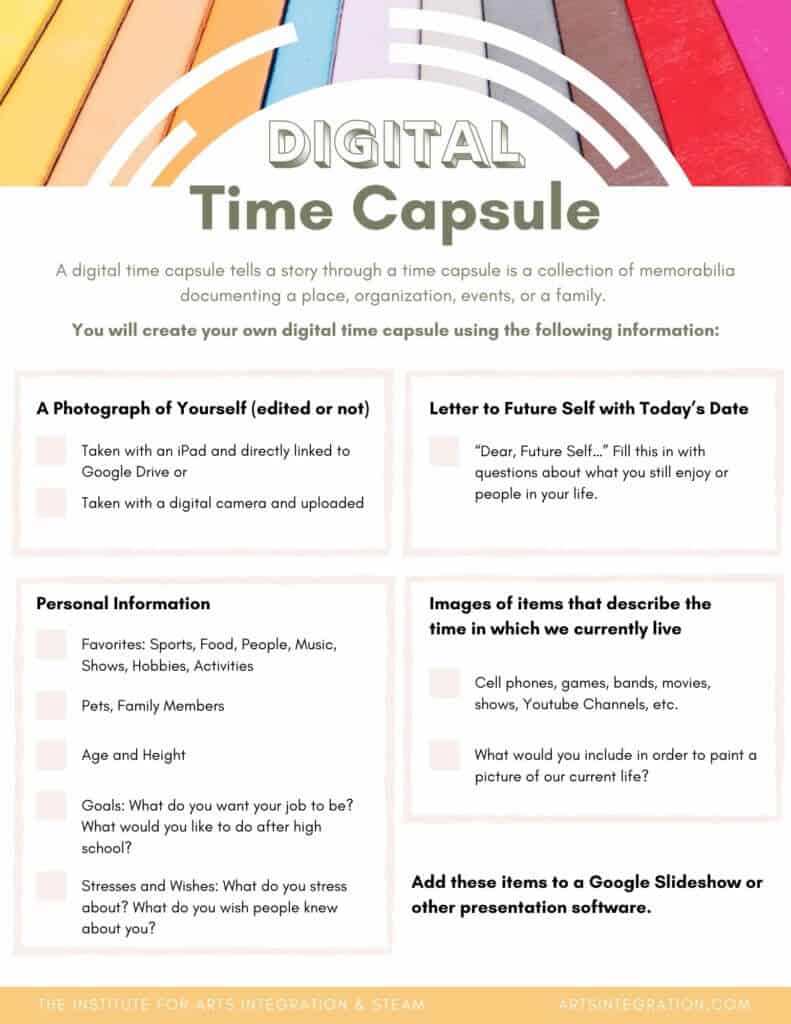This image features a vibrant, multicolored flyer titled "Digital Time Capsule." The flyer serves as an instructional guide on creating a personal digital time capsule, likely intended for a classroom setting. It outlines a project where individuals document various aspects of their current lives through a series of steps. The top portion of the flyer prominently displays the title “Digital Time Capsule” against a colorful banner, with "Digital" in varied tones and "Time Capsule" in black ink. 

The core instructions are well-defined: first, include a portrait of yourself, which can be taken with an iPad and linked to Google Drive or captured with a digital camera and uploaded. Second, write a letter to your future self dated today, addressing current interests, people in your life, and questions about future enjoyment. Third, provide personal information, encompassing favorite sports, foods, people, music, shows, hobbies, activities, family memories, age, height, goals, desired future job, post-high school aspirations, stresses, and wishes. Finally, compile images of items that reflect the current era, such as cell phone games, bands, movies, TV shows, and YouTube channels.

The instructions emphasize adding all these elements to a Google Slideshow or other presentation software. At the bottom right of the flyer, affiliations are noted with the Institute for Arts Integration and STEAM, alongside a website link, reinforcing its educational purpose. This detailed guide not only directs the creation of personal digital archives but serves as a creative exercise in self-reflection and historical documentation.